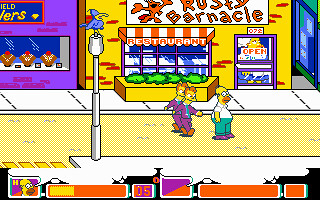This detailed image is a screenshot from an older, retro-style Simpsons-themed video game, reminiscent of Leisure Suit Larry in its graphic quality. In this colorful, 8-bit scenario, Homer Simpson is seen walking down a tan road in front of "The Rusty Barnacle" restaurant, which features a lobster mascot and an "open" sign. Two identical characters in purple suits, complete with blue shirts, red shoes, and orange hair, are chasing Homer from behind with their arms outstretched. To the left of the restaurant, theres’s a purple jewelry store displaying necklaces on mannequins. In the lower bars of the image, a lifeline indicator shows Homer's remaining health at about one-quarter. Additionally, a light post with a bird on top is visible, enhancing the town atmosphere. Homer's outfit consists of a white shirt, blue pants, and purple shoes. The game's score at this point is marked by a number five at the bottom of the screen.